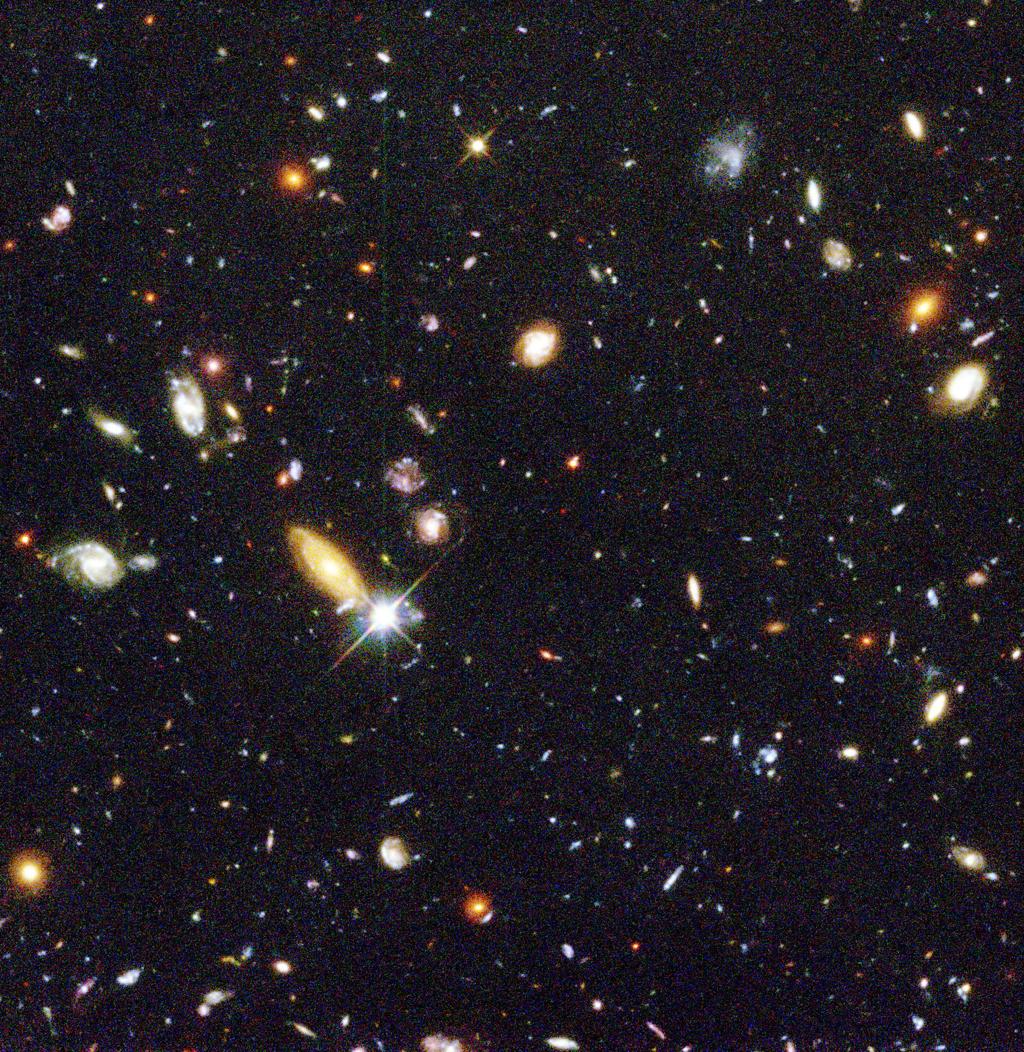A stunning astrophotograph showcasing the vastness of outer space set against a completely black backdrop, resembling a perfect square canvas. The image features an array of hundreds of bright objects, akin to scattered diamonds on black fabric, including swirls of luminescent light that may represent distant galaxies. A particularly bright light towards the middle left of the photo stands out, gleaming like the shiniest diamond under a spotlight. The scene is sprinkled with red, yellow, orange, and light blue hues among a majority of white and light blue dots, simulating stars, comets, or planets. Amidst the multitude of twinkling lights, there are swirling formations on the top right and other areas, adding depth to the celestial panorama. Some formations even resemble asteroids or nebulae. This awe-inspiring image captures the innumerable galaxies suspended in the vast, dark expanse of space, evoking a sense of wonder at the universe's infinite beauty.